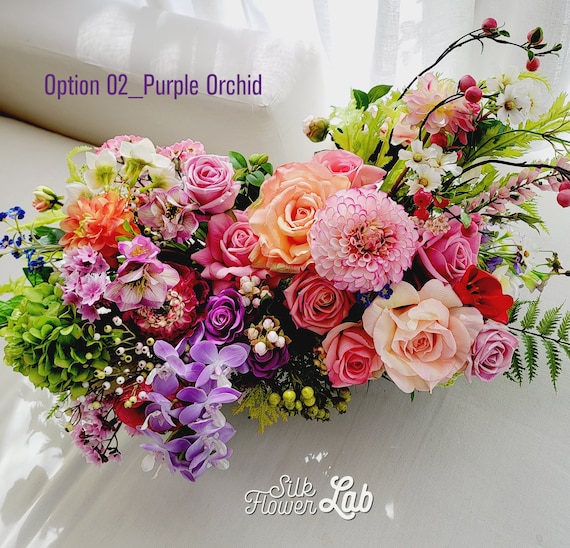This image features a meticulously arranged bouquet of artificial flowers against a gray background. At the top left corner, purple text reads, "option 02_purple orchid," while white text at the bottom center states, "Silk Flower Lab." Dominating the bouquet is a striking purple flower with a white inner core and purple-edged petals, centrally placed. Just above this, there is a large orange rose. To its left, two pink roses and a purple one lie beneath, surrounded by additional purple flowers showcasing a blend of purple and white petals. On the right side, ascending towards the top, green branches terminate in blue bulbs, accompanied by a lush array of green leaves varying from dark to light hues. Some light green leaves extend beyond the frame on the right. Scattered throughout the bouquet are various other flowers in shades of pink, crimson, peach, and blue, as well as small green and red berry-like bulbs attached to stems, adding vibrant touches to the composition.